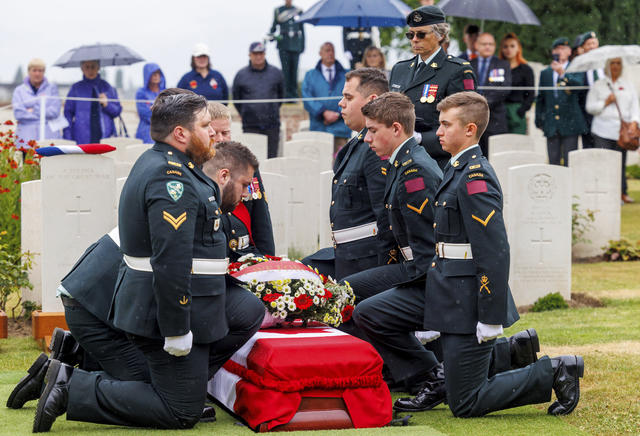This poignant photograph captures a solemn military funeral ceremony for seven World War I soldiers being reburied in Flanders after their remains were discovered during a gas pipeline construction. Five soldiers in army uniforms kneel on one knee beside a casket ready to be lowered into the ground. The casket, draped in a red and white flag and adorned with a floral bouquet, stands out against the backdrop of white tombstones and structures. The scene is somber, with a crowd of mourners, some in suits and raincoats, others with berets and sashes, standing respectfully. Many hold umbrellas, suggesting recent rain despite the clear daytime sky. The image encapsulates a poignant moment of tribute and reverence in a graveyard.